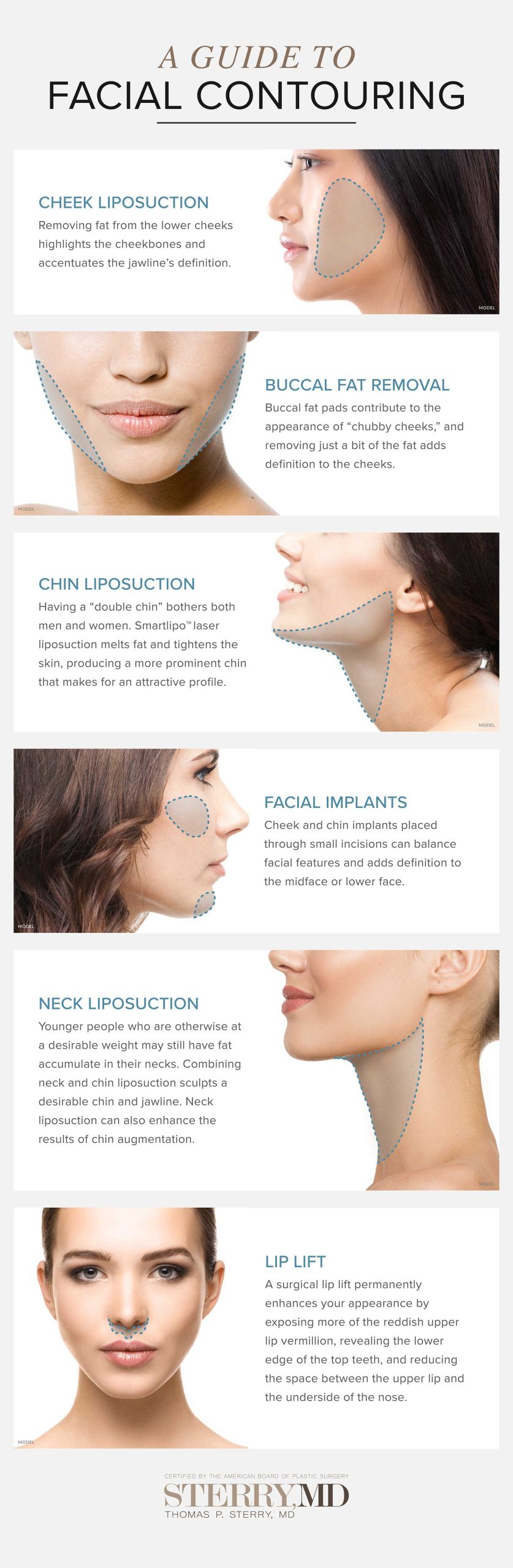This informational image serves as "A Guide to Facial Contouring," featuring a poster with six distinct images highlighting different facial contouring procedures for women. Each image, portraying an outline of a woman's face from either a side profile or a full front view, illustrates specific areas targeted by these procedures. 

1. The first panel, labeled "Cheek Liposuction," outlines the area from the jawline to the upper cheek. 
2. The second panel, titled "Buccal Fat Removal," highlights the section below the cheeks and the bottom jaw.
3. The third panel, "Chin Liposuction," focuses on the chin and upper neck.
4. The fourth panel indicates "Facial Implants," outlining areas on the cheekbones and chin.
5. The fifth panel is about "Neck Liposuction," showing both the upper and lower front neck.
6. The final panel, "Lip Lift," highlights the area under the nose.

The comprehensive guide visually and textually explains each specific facial contouring technique, with the consistent use of women's facial outlines to detail the areas treated.